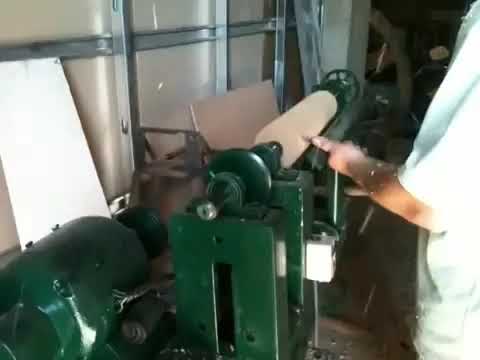The photograph captures a detailed view of a bold green mechanical device, likely a component of an industrial engine or textile machinery, situated in an indoor setting. The machinery features a metallic base and a prominent roller in the middle, around which a cream-colored paper or sheet appears to be wrapped. The machine also has tubes or cylindrical components that resemble large paper towel rolls. Behind the machine, a gray wall is lined with vertical and horizontal metallic silver beams.

On the right side of the device, a person dressed in a short-sleeved white t-shirt is engaged with the machinery, either touching it or pointing towards it. The individual's face is not visible, as the image captures only parts of their body, particularly their outstretched arms. Two such machines are present in the photograph, with one being fully visible and another partially visible. In the background, additional materials can be seen, indicating a cluttered industrial or workshop environment. The scene is well-lit, suggesting it is either daytime or that the room has ample indoor lighting.